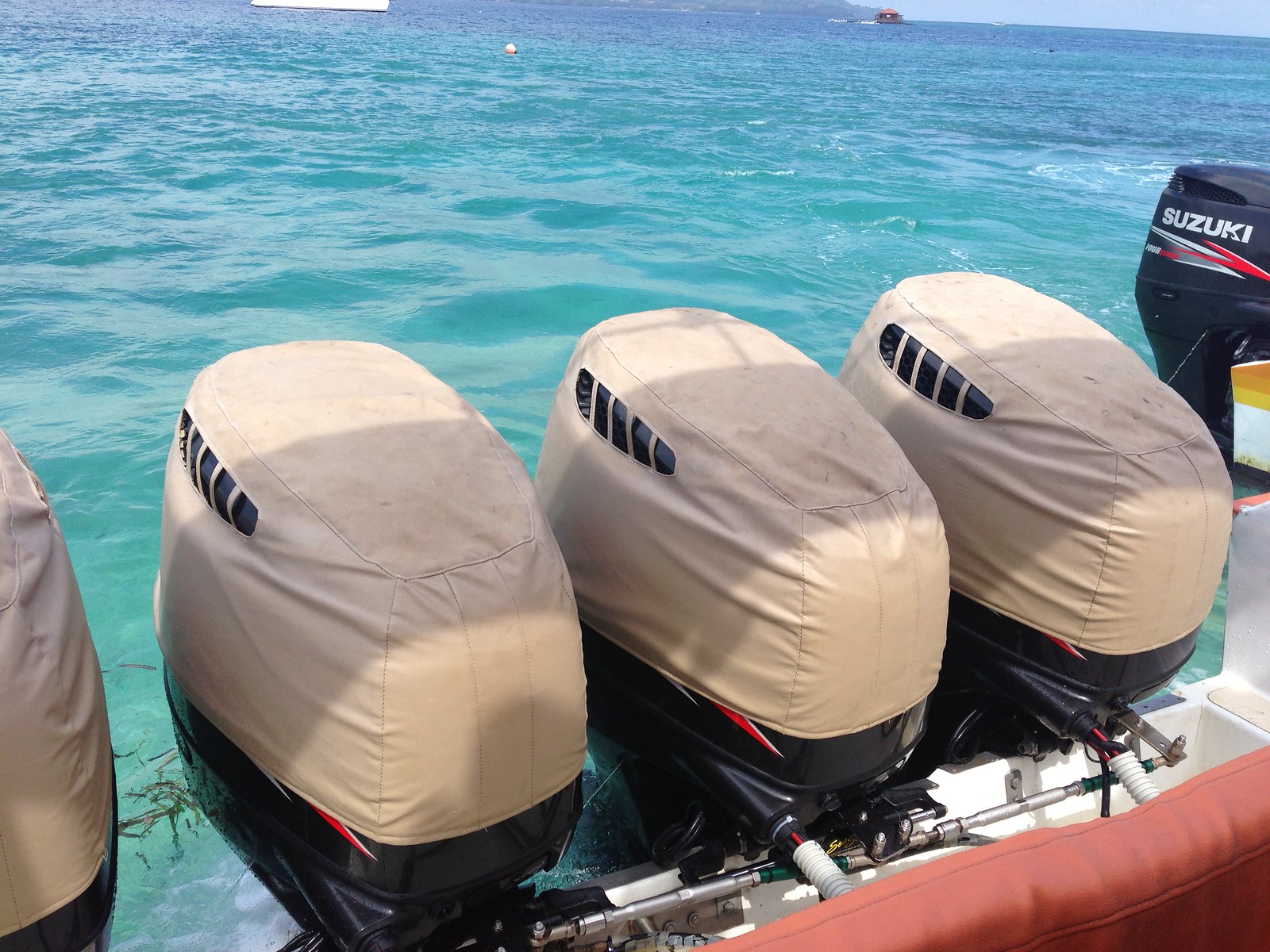This midday photograph captures the back end of a motorboat on a calm, light blue ocean. Prominently featured are four large motors, each partially covered with beige protective covers, while the actual engine covers are black. The logo on the motors is obscured. In addition to the main motors, there is a smaller kicker motor, specifically a Suzuki, towards the right side, also with a cover. A red padded backrest is visible as well. The ocean appears tranquil, with its blue-green waters slightly rippling. In the distant background, a small buoy is noticeable, and another boat can be vaguely seen. The sky, just peeking into the frame, is clear and blue.